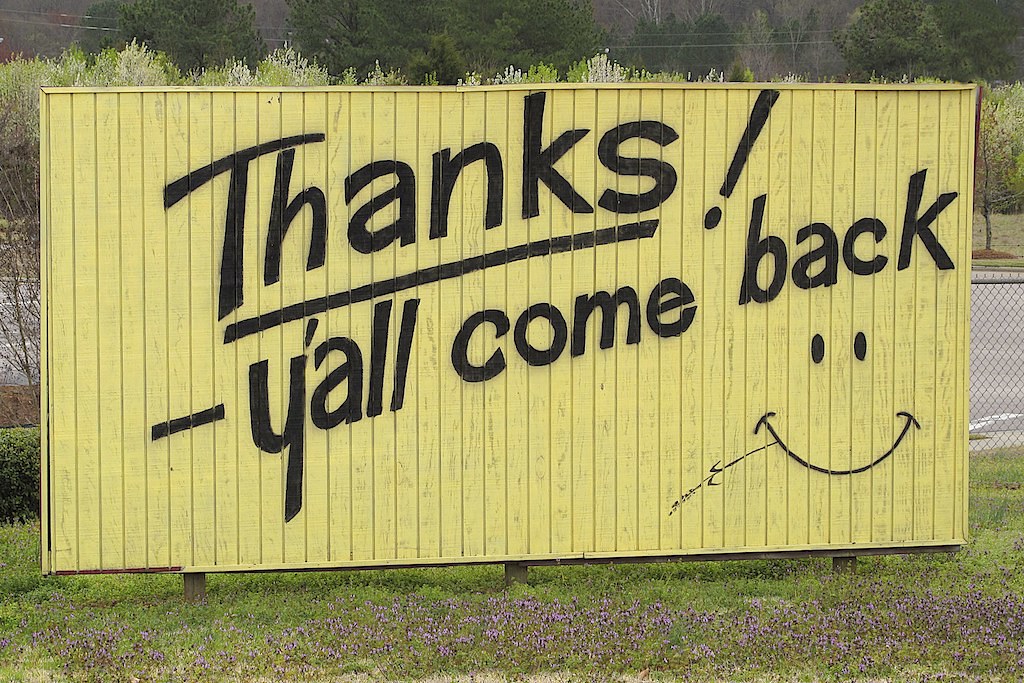The photograph captures a detailed scene with a prominent sign in the foreground. The sign is a rectangular, horizontal structure composed of light gold vertical slats. In bold black lettering, it cheerfully reads "Thanks!" with an underline, followed by a casual "Y'all come back!" signed off with a playful smiley face. The smiley features two eyes and a grin, with a piece of grass sticking out from the left side of its mouth.

Below the sign, green grass flourishes, interspersed with clusters of purple flowers at ground level, adding a touch of natural beauty. Moving backward, a wire fence delineates the area, possibly enclosing a blacktop surface that remains indistinct—perhaps a playground or a path. In the mid-ground, a row of sapling trees catches the eye, their light green leaves adorned with delicate white blossoms. The tips are mostly visible, except for the tree on the far right which is more prominently exposed.

Far in the background, a mixed setting emerges with darker, shadowy elements accompanied by clusters of green trees, providing a vibrant and lush backdrop that is not blurred, contributing depth to the overall image.